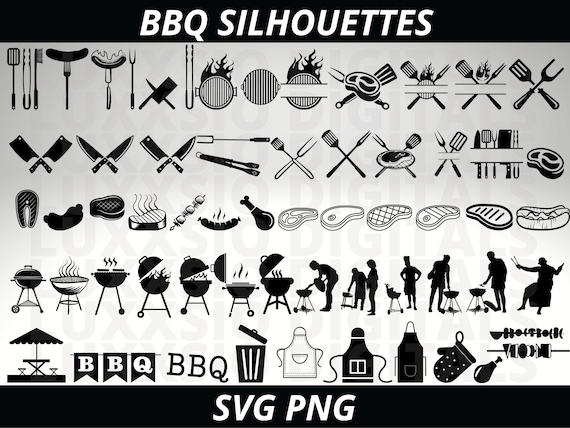This landscape-oriented image showcases an assortment of barbecue-themed clipart, set against a grey background with prominent black bars at the top and bottom. The top bar features white italicized uppercase text reading "BBQ Cinderheads," while the bottom bar displays "SVG" and "PNG" in similar fashion. The layout is composed of five rows of various icons and silhouettes that emphasize barbecue tools, settings, and accessories, each neatly arranged for visual clarity.

In the top rows, the icons display a range of cutlery including forks, tongs, ladles, spatulas, and various knives, along with symbols of grill marks and fire. The middle rows feature an array of meat products such as steaks, hot dogs, shish kebabs, and chicken drumsticks. Further down, the icons illustrate different styles and sizes of grills, often accompanied by the silhouettes of individuals cooking or standing nearby, equipped with aprons and mittens.

In the bottom row, additional picnic essentials are depicted, such as an umbrella for a picnic table, a park bench, a trash can, and signage with the word "barbecue." Overall, the detailed clipart elements in black and white create a cohesive visual representation ideal for illustrating barbecue contexts in digital formats such as SVG and PNG.